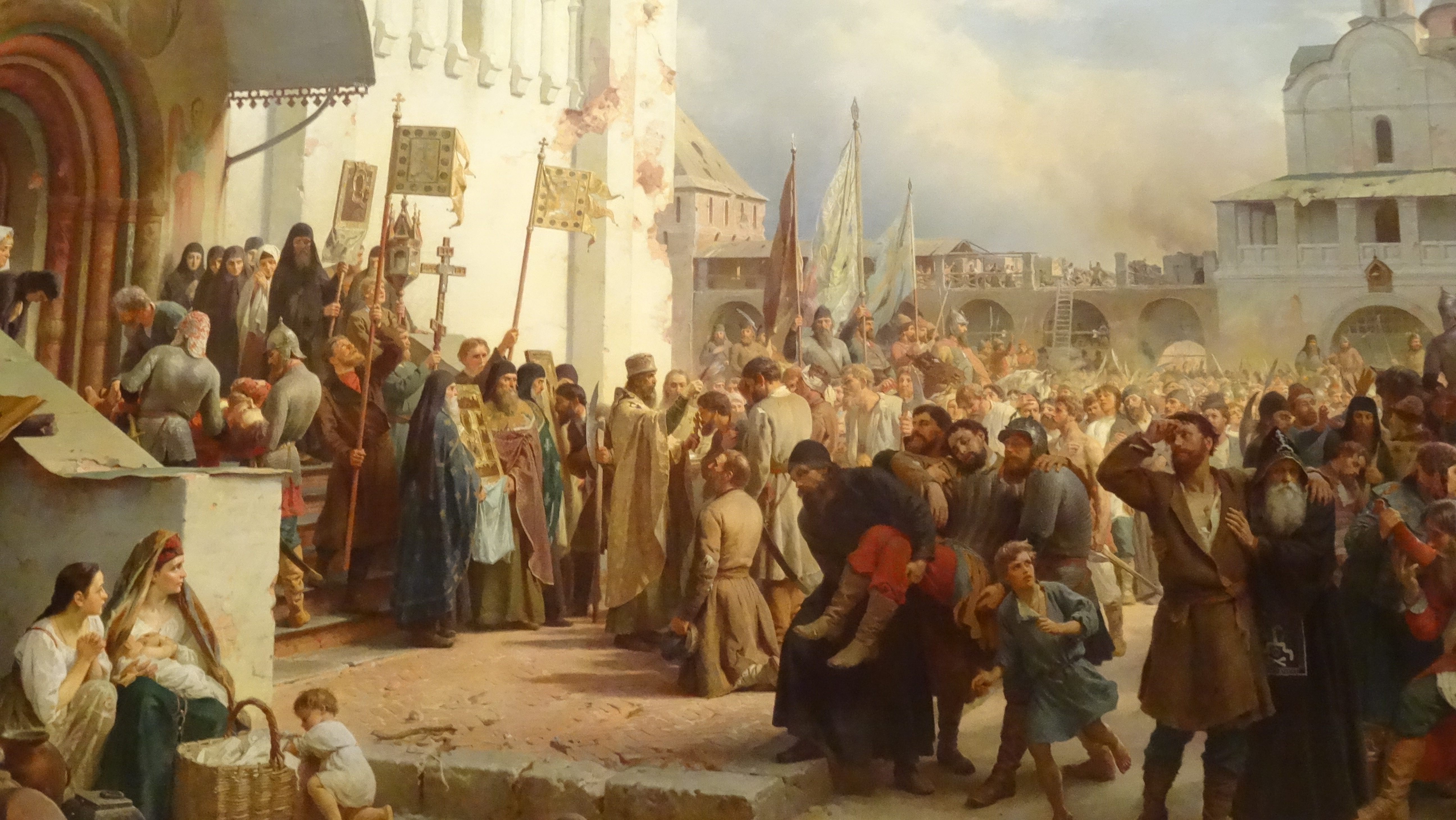The image is a highly detailed, photorealistic painting capturing a bustling scene outside the entrance of an elaborate church. The church features an arch-shaped opening and several steps leading up to it. In the foreground, on the right side of the church, a large crowd has gathered, filling the street. On the left side, at the church entrance, numerous people dressed in long robes and headscarves stand solemnly, some holding a square flag adorned with many small patterns and others holding crucifixes. At the forefront of this group, a priest is seen addressing the people gathered. Near the church’s steps, there appears to be a person being carried—possibly by guards or officials—which has created a considerable commotion among the crowd.

Amidst the throng, clergy members and possibly knights or officials can be seen, adding to the sense of a significant event or ceremony in progress. Additionally, off to the left side in the foreground, women are seated on a step, with one woman holding an infant and another with a baby in a basket playing nearby. Surrounding the scene are various buildings, hinting at a town square setting, all under a cloudy blue sky. This intricate painting captures the intense emotions and intricate details of a community in the midst of an important and possibly distressing public gathering.